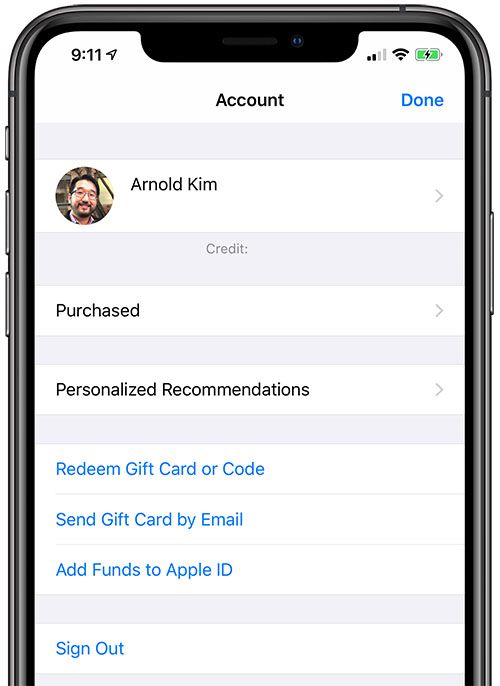The image depicts a dark silver cell phone with a visible interface, highlighting various details. The screen primarily shows a white background with alternating light gray lines displaying 9:11 AM. Indicators for cellular signal, Wi-Fi connection, and a green, charging battery icon are positioned at the top. At the screen's top center, the word "Account" is displayed, and to the right, in blue, reads "Done."

A profile section features the name "Arnold Kim" with a small photo of an Asian man with black hair, a beard, and a mustache, having a light pinkish-tan complexion. This profile section includes a right-pointing arrow and is set against a gray background. Below this, a series of options are presented on alternating white and gray bands:

1. "Credit;" is in the middle, followed by "Purchased" in black text with a right arrow on a white band.
2. "Personalized Recommendations" in black with a right arrow on a white band follows a gray band.
3. "Redeem Gift Card or Code" in blue text on a gray band.
4. "Send Gift Card by Email" in blue text on a gray line.
5. "Add Funds to Apple ID" in blue text, followed by another gray band.
6. Finally, "Sign Out" in blue text on a white band at the bottom.

The image cuts off just below this point, leaving the bottom of the phone and the page out of view.